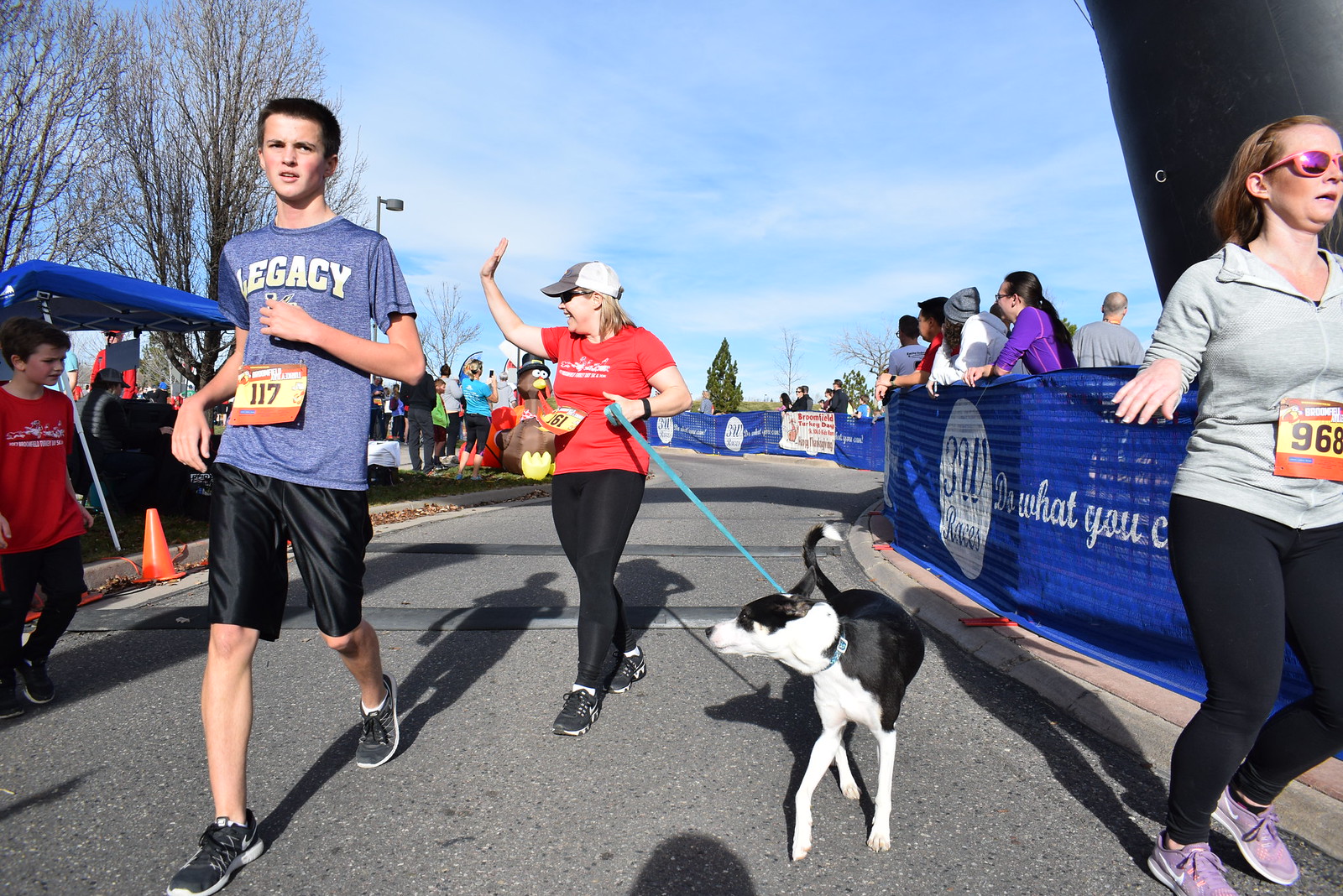In this vibrant and engaging photograph, we find ourselves immersed in the bustling atmosphere of a marathon nearing its finish line. The scene captures over 200 participants, each donning numbered apparel, ranging from a young man in a blue shirt and black shorts with the number 117, to a woman sporting number 968, clad in a gray sweater, black tights, and purple shoes.

A prominent figure in the image is a lively woman wearing sunglasses, a white cap, a red shirt, and black leggings. Waving enthusiastically to the crowd, she radiates joy and energy. Notably, she is accompanied by a medium-sized white and black dog on a leash, hinting at the possibility that she might be visually impaired, as she wears the number 161.

The lively marathon is further accentuated by the cheering spectators lining both sides of the route, their excitement adding to the spirited ambiance of the event. The sky overhead is refreshingly cloudy, but devoid of any threatening rain clouds, contributing to the perfect conditions for this athletic event. This snapshot captures a moment of shared determination and communal celebration, with runners and onlookers alike participating in the collective experience of the race.